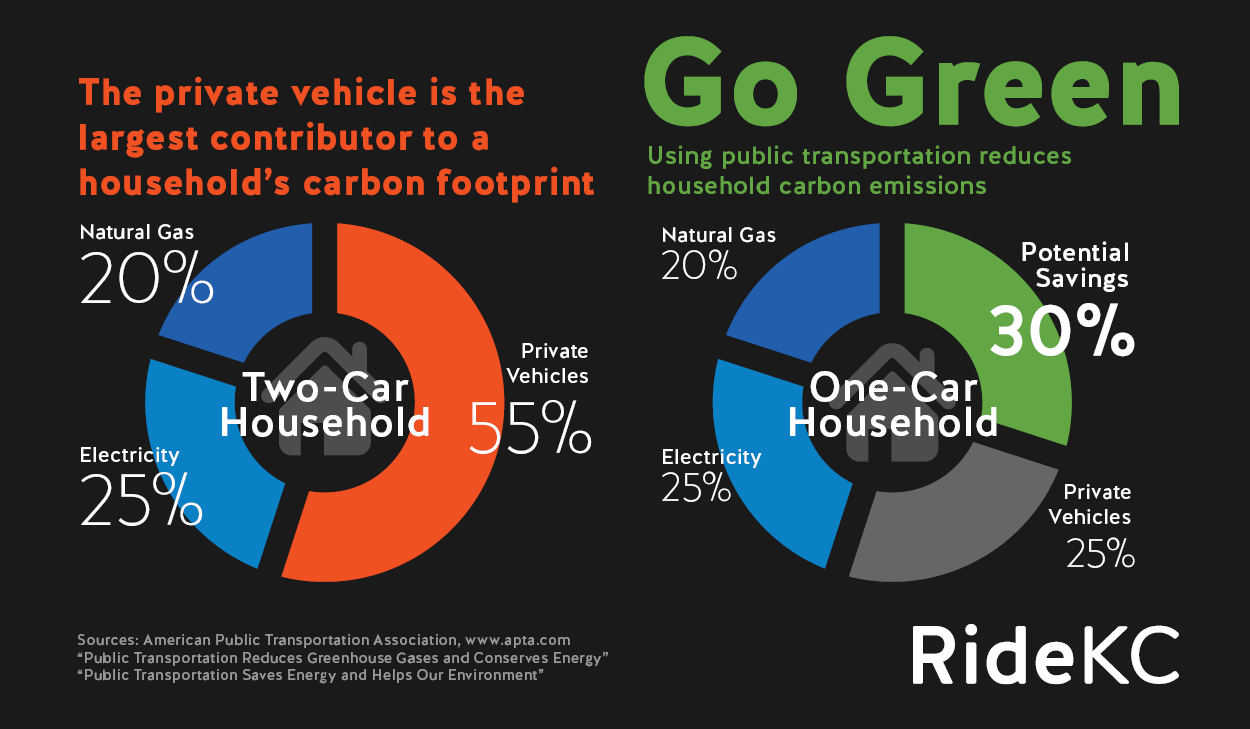The "Go Green" poster promotes the environmental benefits of using public transportation. It urges audiences to "Go Green" and stresses that "using public transportation reduces household carbon emissions." The poster highlights that "the private vehicle is the largest contributor to a household's carbon footprint," displayed prominently in red and orange text. 

On the left side, there is a donut pie chart illustrating the carbon footprint of a two-car household. This chart shows that private vehicles account for 55% of the emissions, while electricity and natural gas contribute 25% and 20%, respectively. In comparison, the right side features a donut pie chart for a one-car household, indicating potential savings of 30%. In this scenario, private vehicles contribute 25%, electricity 25%, and natural gas 20% to the household's carbon footprint. Each section of the charts is color-coded in blue, dark blue, green, and gray, with percentages labeled in white font. 

The chart captions emphasize the environmental impact reduction from private vehicle use to public transportation. The poster concludes with the "RideKC" logo in the bottom right corner and attributes data sources to the American Public Transportation Association (www.apta.com). An asterisk notes that public transportation helps reduce greenhouse gases and conserve energy. The entire infographic is set against a black background, enhancing the contrast and visibility of the information.